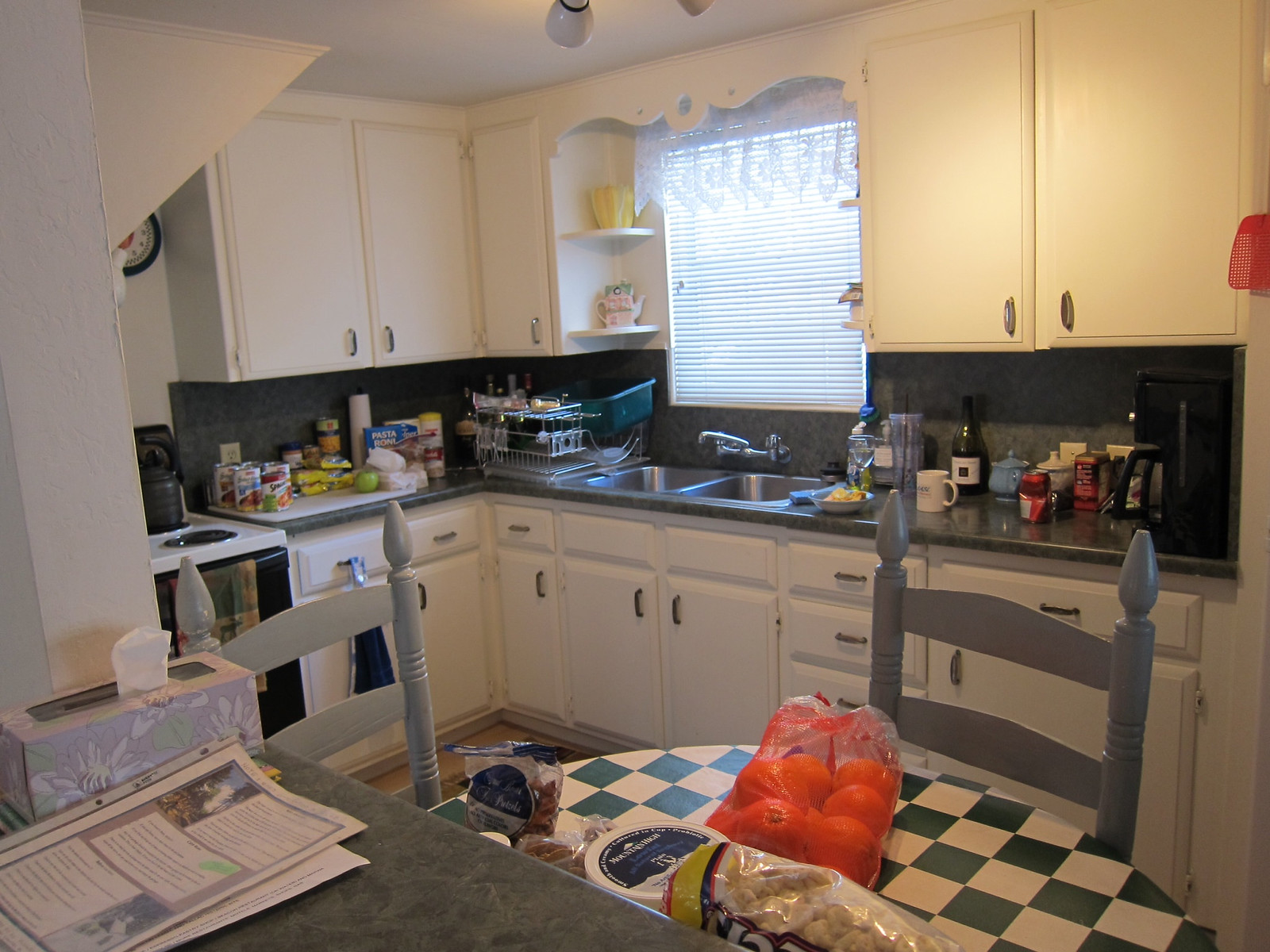The image captures a meticulously detailed view of a kitchen from a slightly elevated angle. The kitchen is furnished with white upper and lower cabinets that provide a classic and clean look. The countertop is a polished gray marble that pairs harmoniously with the kitchen's gray tiled backsplash, adding a touch of modern elegance.

To the left of the cabinets, there is a white stovetop with a black oven door. In front of the stove, there's a collection of food items, including several canned goods—of which one appears to be spaghetti or SpaghettiOs. Alongside the cans, there are piled bags of food, a lone green apple, a blue box labeled "PastaRoni," and a roll of paper towels.

Adjacent to these items sits a dish rack, followed by a sleek, stainless steel double bowl sink. To the right of the sink, additional culinary items are spread out, featuring a bottle of wine, a bowl that seems to hold fruit (though slightly out of focus), a crushed aluminum can, and a coffee maker.

In the image's foreground, there is a round kitchen table draped with a black and white tablecloth. The table is surrounded by gray wooden chairs. On the table sits a bag of oranges and several other indistinct food items in bags, adding to the room's lived-in feel. The overall scene is a blend of utility and comfort, indicative of a kitchen that's actively used and well-loved.